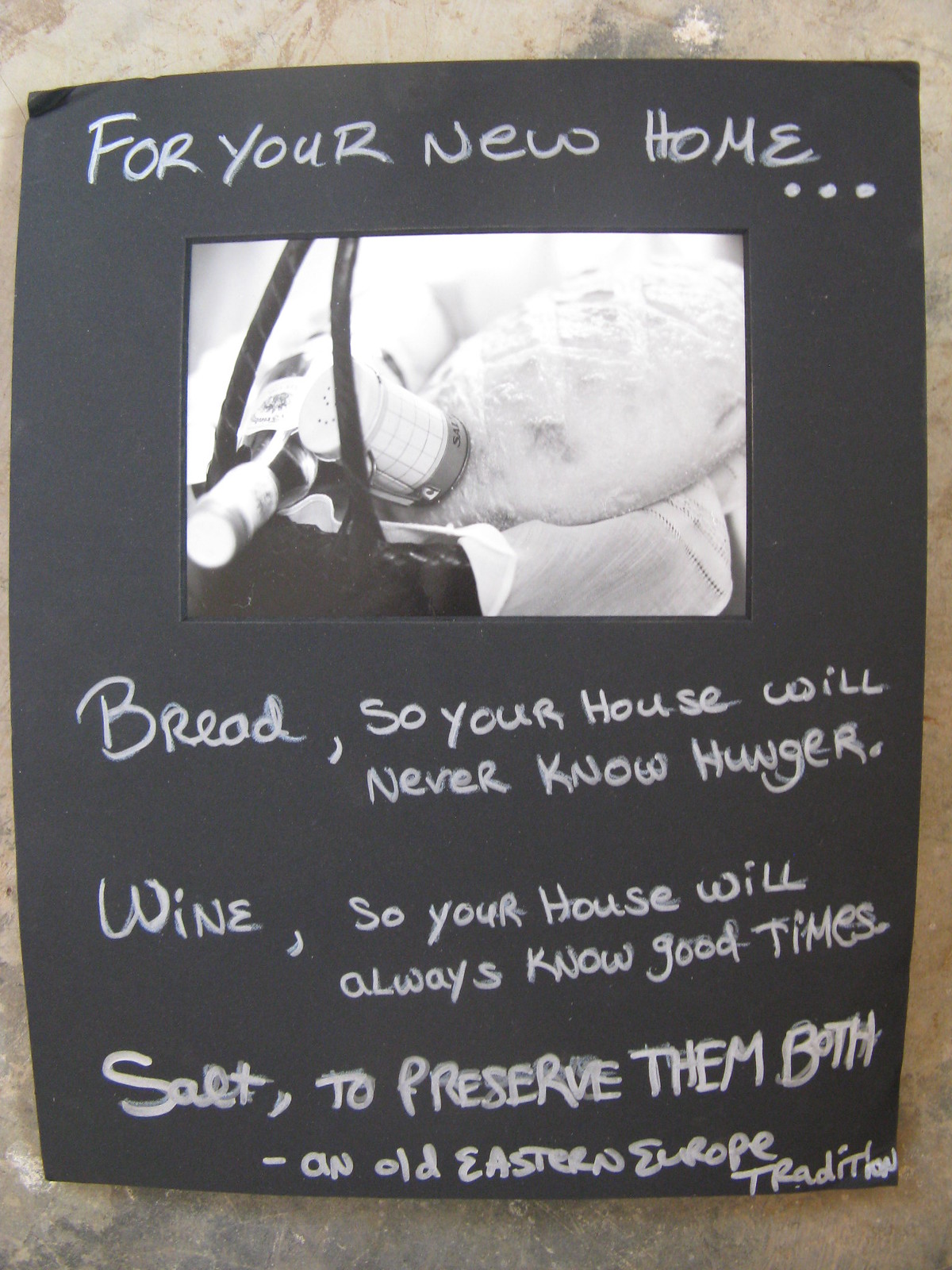This black and white image appears to be a homemade card, presented on what looks like black paper stock, possibly resembling a blackboard, with handwritten white text, likely written in chalk or ink. The background is black and appears to be taped up, slightly bowed out in the middle. At the top, the card reads "For your new home..." in white text. Beneath this, there's a black and white photo of a basket containing bread, wine, a salt shaker, and a cloth draped over the edge. Below the image, white text states "Bread, so your house will never know hunger. Wine, so your house will always know good times. Salt, to preserve them both. An old Eastern Europe tradition." The entire presentation harks back to an old Eastern European tradition, captured thoughtfully in this handmade card.